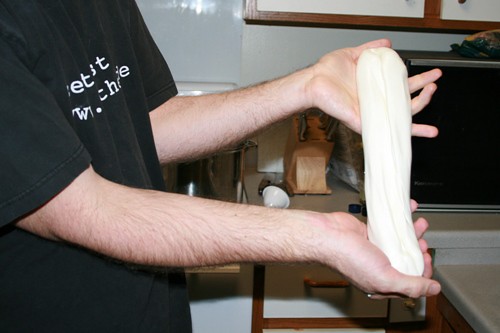A man with a fair complexion is depicted in this detailed kitchen scene, focused on preparing dough, likely for bread or pizza. He is standing on the left side of the image, stretching a light beige piece of dough between his hands, with his left hand positioned higher than his right. He is wearing a black shirt with white lettering, though it's unreadable due to the side profile and wrinkles. His arms, which are noticeably hairy up to the elbows, are fully extended, creating ripples in the dough. In this well-equipped kitchen, the countertops are grey marble supported by dark brown wood, complemented by similarly styled cabinetry. A microwave is positioned on the counter amidst various cooking supplies, with a bag perched atop it. To the left of the microwave, there’s a light brown wooden knife rack with silver-handled knives and extra slots. Another notable detail includes a large steel cooking pot partially visible between the man's arms. The floor appears to be solid grey, and the overall setting is clean and organized, emphasizing the man’s engaging dough-stretching activity.